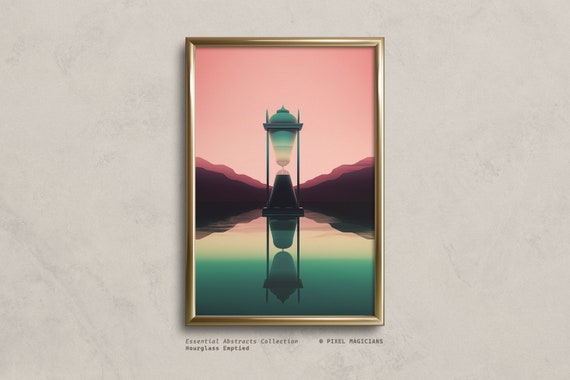The image depicts a painting hung on a wall that features a marble-like pattern, characterized by its white color interspersed with grayish veins. The painting is encased in an ornate gold frame, enhancing its regal appearance. The artwork itself is abstract, portraying a surreal hourglass against a pink sky. The hourglass, fashioned in teal and resembling a pair of vases or acorns, showcases sand flowing into three sections, with reflections suggesting water at the base. Subtle hues of mauve, green, and darker maroon hues enrich the scene, adding depth and mystique. Below the painting, a plaque reads "Essential Abstracts Collection," "Hourglass Emptied," by "Pixel Magicians," affirming its placement in a curated collection.